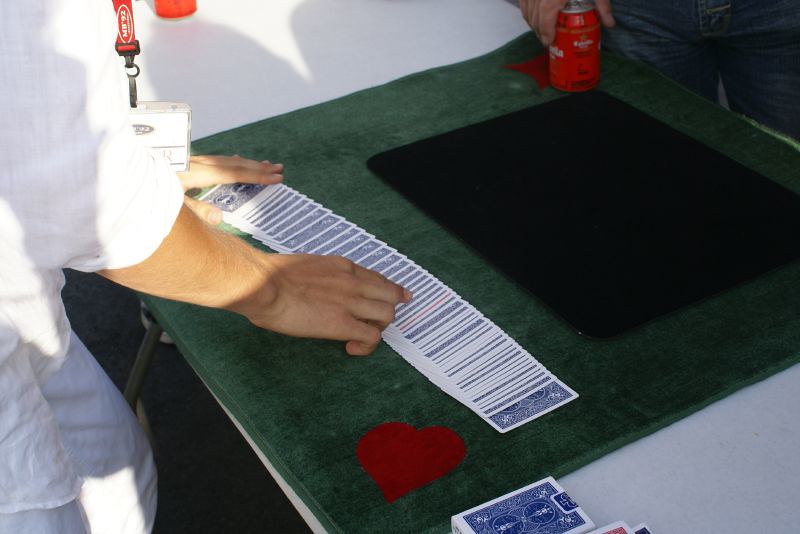A detailed scene unfolds as a card dealer expertly lays out a deck of blue, standard design cards on a green felt table cover, preparing for a game of blackjack. To the dealer's right is a box of cards, indicating readiness for extended play. The dealer, dressed in a white shirt with three-quarter sleeves tastefully rolled up, focuses on the task at hand. In the shot, only the fingers of another player are visible, holding an orange can of beer, suggesting a casual, relaxed atmosphere. The arrangement and setting hint at an engaging night filled with card games, be it a round of blackjack or perhaps a captivating card trick to kick off the evening.